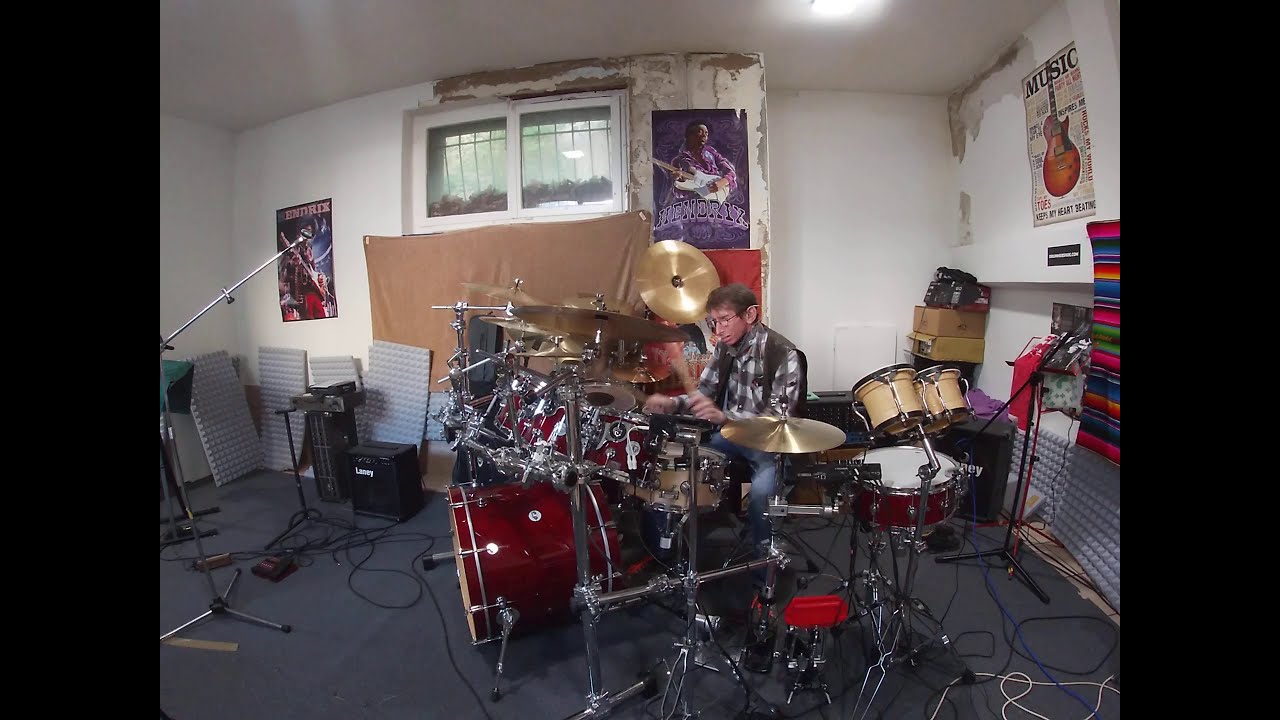This is a detailed photograph of an indoor musical room dominated by a central drum set. The metallic red drum set with silver stands is being played by a person sitting on a stool. The drummer is dressed in blue jeans, red and gray shoes, a white and black plaid shirt topped with a black vest, and glasses. The drumsticks in their hands appear slightly blurred, indicating motion. The walls of the room are primarily painted white, though parts of the paint have chipped away, revealing a brown base in several corners and edges. Scattered across the room are various musical instruments, speakers, and a tangle of wires running toward the front. A gray floor sets a neutral backdrop for the setup. Several music-related posters decorate the walls, including a prominent Hendrix poster, a guitar poster labeled 'music', and another featuring a musician with a guitar. Additionally, the room has three windows—one on the top center, one on the left, and one on the right, allowing natural light to filter in. A microphone on a stand and large speakers on the floor are also visible, contributing to the room's vibrant musical atmosphere.